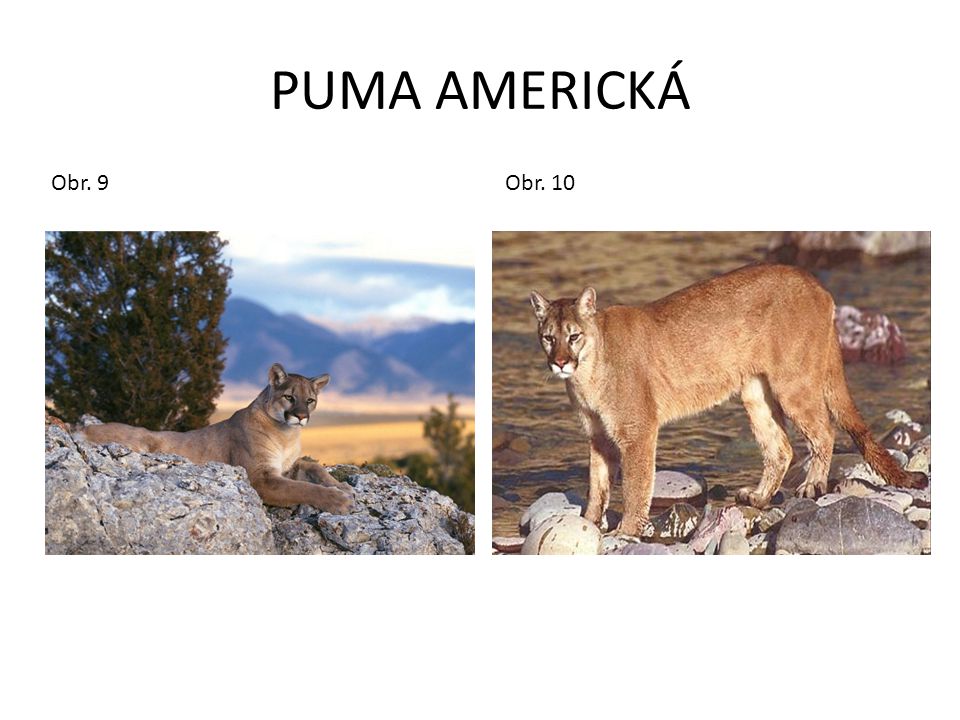The image consists of two photographs of pumas, seemingly excerpted from a guidebook depicting these majestic animals. At the top in bold, black capital letters, it reads "Puma América" (with América spelled as "América" including an accented "A" and a prime symbol next to the "C").

In the left photo (captioned "OBR.9"), a puma is seen laying on its stomach on a rocky cliff, its head raised and facing the camera. A tree is positioned to its left with a vast, mountainous landscape unfolding in the background. The sky above the distant hills appears to be either during sunrise or sunset, with hues of blue and pink mixed with golden-brown valleys in the distance.

The right photo (captioned "OBR.10") depicts a puma standing on rocky terrain before a stream, also facing the camera. This scene highlights a rugged, water-adjacent landscape, emphasizing the cougar’s alert and watchful stance with its tail lowered.

The combined focus of these images effectively portrays the versatile habitats of pumas in the Americas.